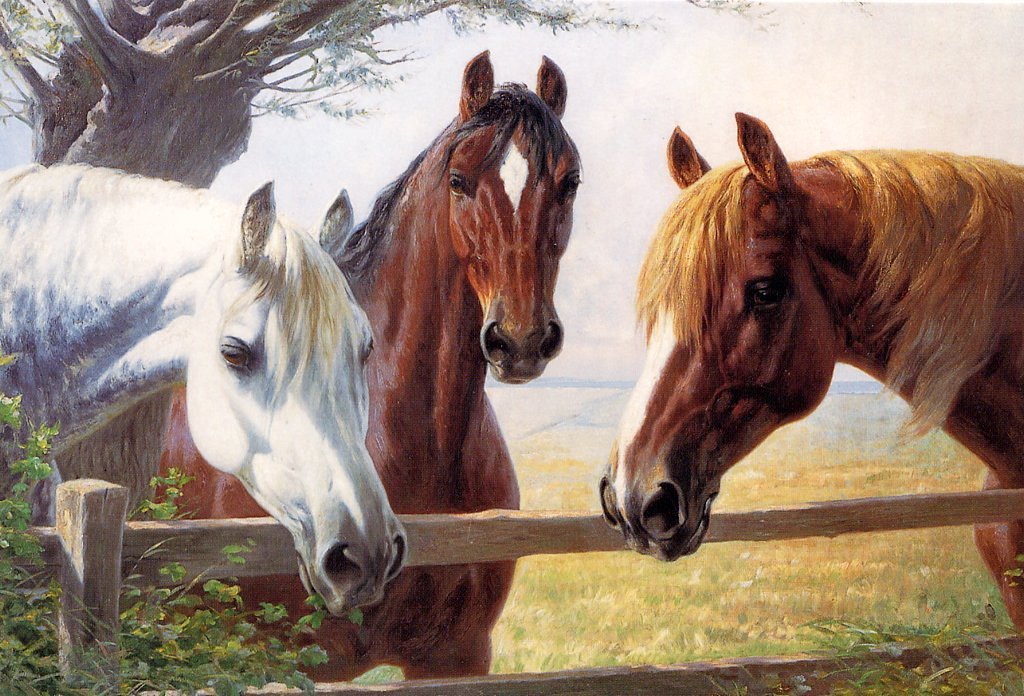The detailed image showcases a color oil painting of three horses, rendered with fine detail and an impressionistic touch. Positioned behind a split-railed, light grey wooden fence, these majestic creatures gaze out serenely. On the left is a predominantly white horse with a white mane, accentuated by a few strands of tan or golden hair around its eyes and nose, which gently rests on the fence. The middle horse, with a rich brown coat, features a distinctive white diamond on its forehead and a black mane cascading from behind its ears. The rightmost horse, slightly more chestnut in hue, has a striking white line running down its face and a fluffy golden mane that drapes over its neck. In the background, the painting features a foggy or misty white sky, and a grey tree with a few small, wispy leaves in the upper left corner. The scene transitions into a large open field with slightly browned grass, indicative of a summer landscape. Adding to the pastoral setting, a green bush grows through and along the fence in the bottom left corner.